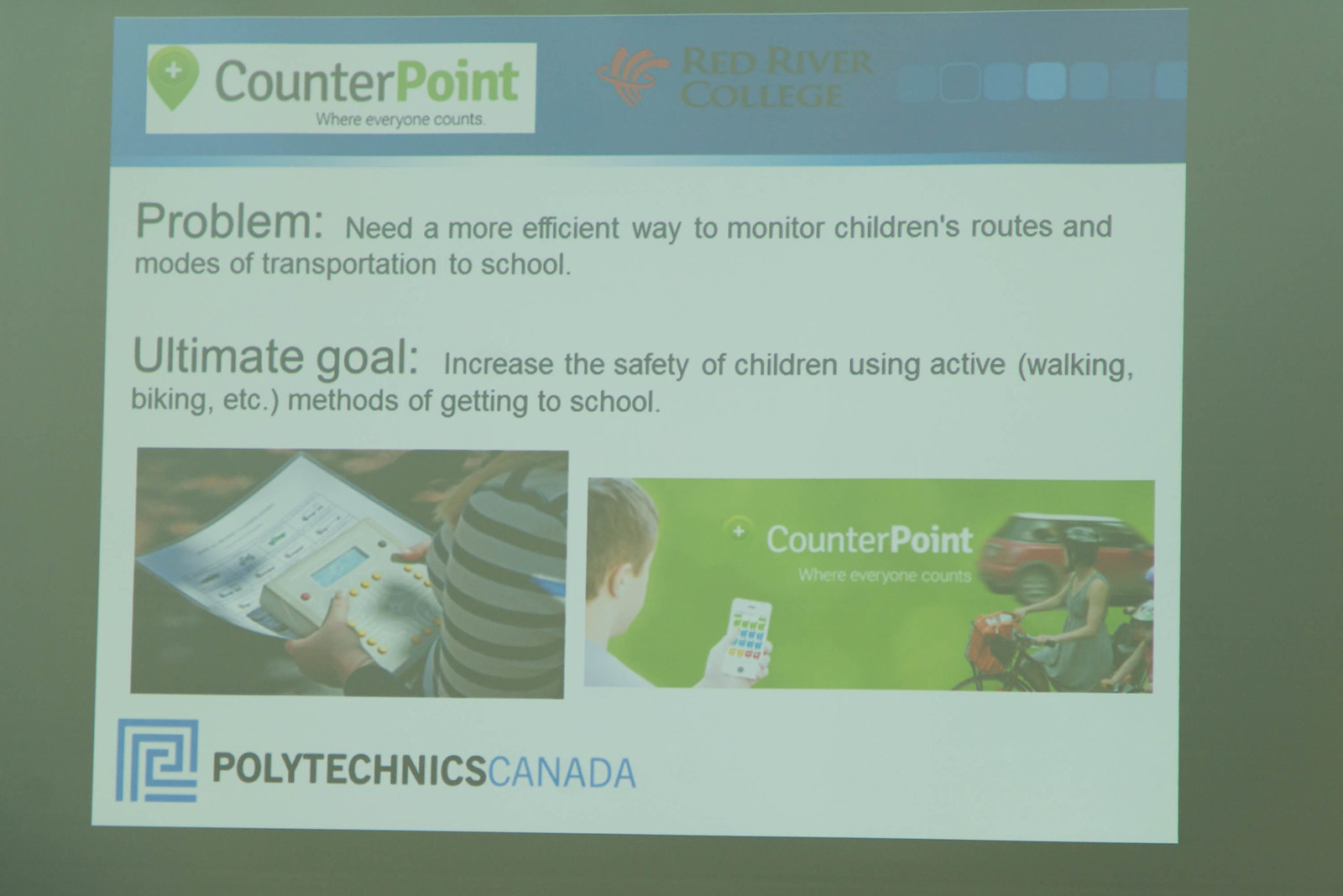In this image, there is a close-up photograph of what appears to be a dimly lit and slightly unfocused PowerPoint presentation slide. The top section of the slide features a blue rectangular strip extending horizontally, with a thinner white rectangular strip to its left bearing the text "Counterpoint, where everyone counts." The word "Point" is highlighted in green. To the right of this, in green text, it says "Red River College." Below this, a row of seven small squares, each in varying shades of blue, runs horizontally.

The main body of the slide has a white background with text that reads, "Problem: need a more efficient way to monitor children's routes and modes of transportation to school." Below this, another section labeled "Ultimate Goal" reads, "increase the safety of children using active (walking, biking, etc.) methods of getting to school." 

Two photographs are positioned side-by-side beneath this text. The left photograph depicts the shoulders of a girl holding a device that resembles a calculator. The right photograph has a green background and shows three elements: someone holding a phone, another person on a bike, and a red car in the background. The text "Counterpoint, where everyone counts" is visible in this photograph.

In the bottom left corner of the slide, the text "Polytechnics Canada" is displayed. The image as a whole has a slight transparency and a foggy look, giving it a somewhat faded appearance. It seems like a photograph taken of the digital screen rather than a direct screenshot.